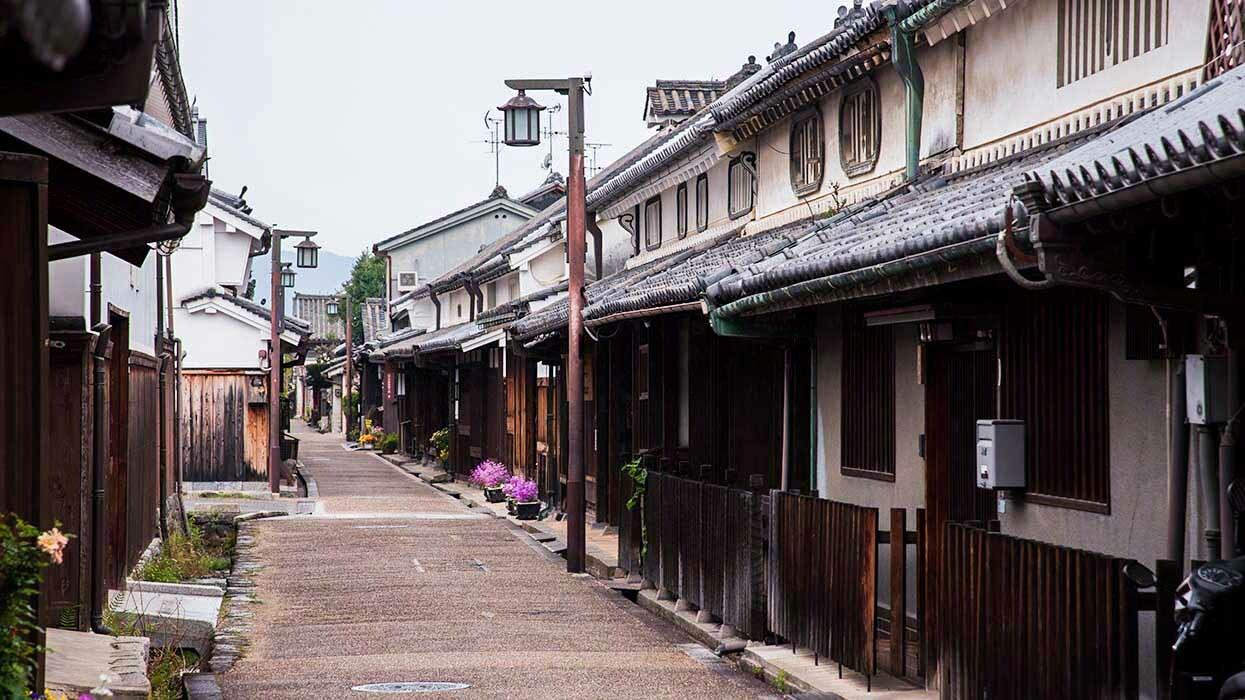The image depicts a picturesque, pedestrian-friendly pathway lined with connected residences, resembling row homes or villas. The central pathway, made of beige concrete or asphalt, is framed by two distinct rows of buildings. On the right, the structures are uniform, featuring beige exteriors with green-gray roof overhangs and upper floors. On the left, the homes are more varied, with one appearing white and another brown. Both sides are adorned with elements of rustic charm, such as brown picket fences, possibly made of wood or iron, and potted plants bursting with purple, yellow, and pink flowers. Streetlights, reminiscent of antique lanterns, dot the pathway, enhancing the scene's quaint, almost idyllic feel. The sky is blue, with distant gray mountains and green trees providing a serene backdrop. The architecture, especially the roofs, suggests an Asian influence, though the exact location remains unspecified. No people are visible in the image, lending a tranquil, undisturbed quality to the residential area.